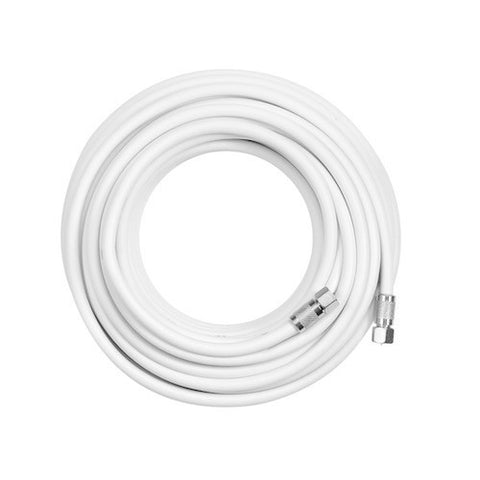This image is a detailed product photograph showcasing a long coaxial cable. The white cable is meticulously coiled into a tight, perfect circle. Each end of the cable features a silver metallic tip, complete with a six-sided screw fitting for easy attachment, likely to a socket or device. Surrounding the screw fitting is a washer and a thread for finger grip, adding to its functional design. The coiled nature of the cable suggests it is very long, with multiple layers visible within the circle. The entire setup rests on a bright, white, and transparent background, which enhances the pristine and clean appearance of the white coaxial cable, making it ideal for transmitting cable TV signals.